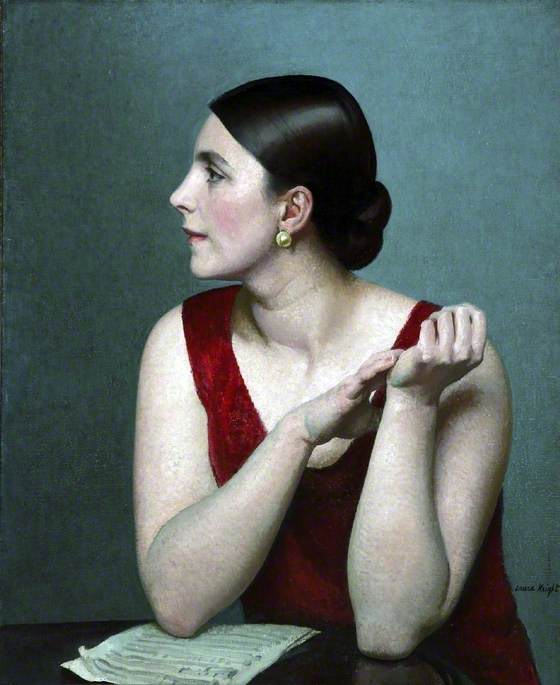A highly realistic painting portrays a young European-Caucasian woman seated at a round, black table with her elbows resting on it. The nuanced background transitions from a lighter bluish turquoise gray on the right to a darker grayish green on the left. At the bottom of the composition, the edge of the table is adorned with two pieces of paper, likely sheet music. The woman, dressed in a red velvet-like dress with thick straps, sits with her elbows atop the table, her right elbow resting on the papers. Her right hand gently clasps her left hand, which is positioned near her shoulder. Her appearance is further accentuated by very pale skin, a sleek black bun, red lipstick, and a large, thick golden earring. She gazes thoughtfully to the left, revealing a profile view of her face. The intricate details and lifelike quality of the painting, along with its subtle background shading, make it difficult to distinguish whether it is indeed a painting or a photograph. A small, indecipherable signature is present in the lower right corner, adding a final touch of authenticity.